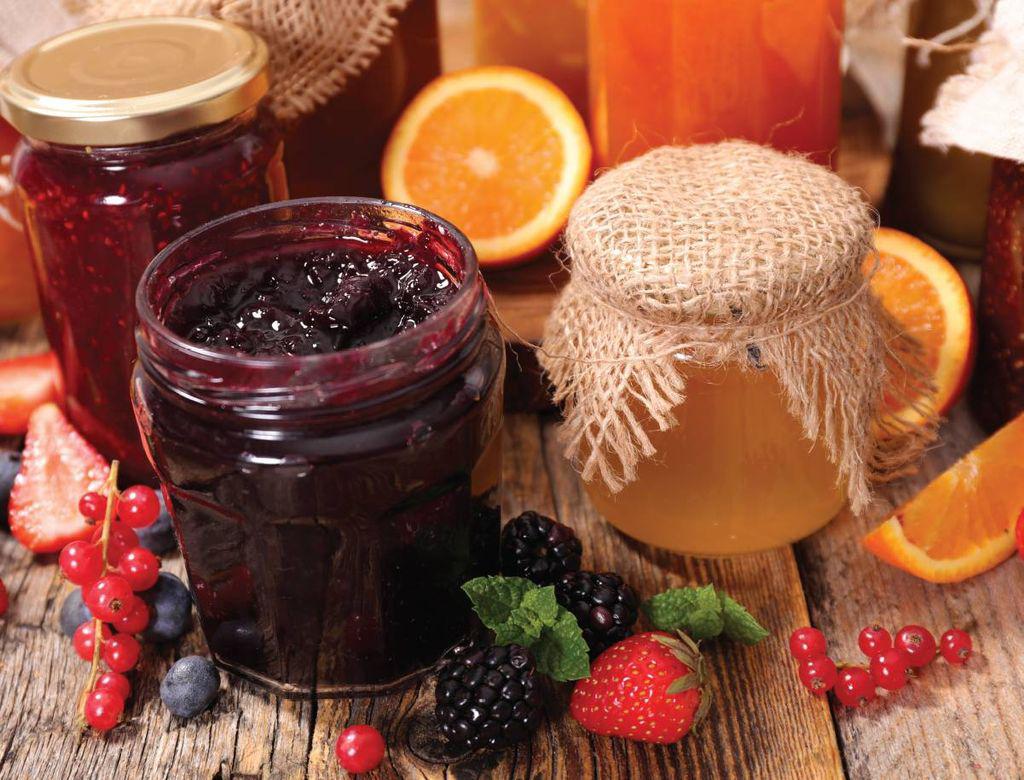The photograph showcases an array of homemade jams and jellies arranged artfully on a rustic, gray-colored wooden table. The focus is on three glass jars in the forefront. One of these jars is open and appears to contain a dark berry jam, possibly blueberry or cranberry. Another jar has a gold lid and is suspected to hold strawberry or raspberry jelly. The third jar, capped and adorned with a burlap cover, likely contains orange marmalade. Additional jars are visible in the background, though their contents are indistinct. Scattered around the jars are fresh fruits that hint at the jams' flavors, including strawberries, blueberries, blackberries, oranges, and small red berries. The table is also accented with slices of cut oranges, enhancing the vibrant, homemade feel of the display.